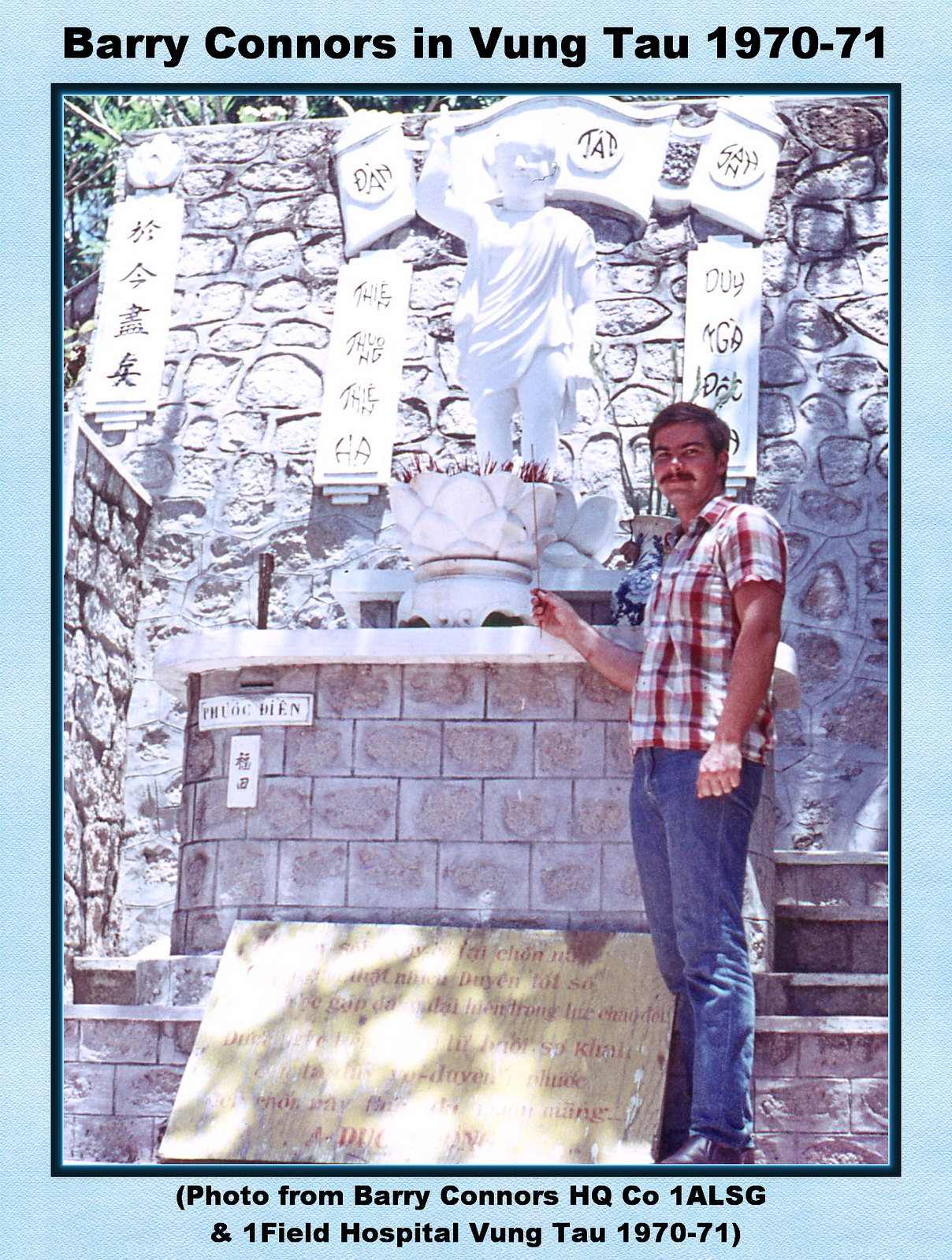This rectangular photograph, surrounded by a light blue matte with a thin black inner border, depicts a man identified as Barry Connors in Vung Tau, 1970-71. At the top of the image, the label reads: "Barry Connors in Vung Tau, 1970-71," and at the bottom, it says: "photo from Barry Connors, HQ CO 1ALSG and Onefield Hospital, Vung Tau, 1970-71." Barry Connors, a young man possibly in his 30s with short dark hair and a mustache, stands smiling directly at the camera. He is dressed in a short-sleeved, red and gray plaid shirt, blue jeans, and brown shoes. Beside him is a small statue of a cherub-like boy with one hand raised in the air, situated on a circular pedestal. This statue, part of a concrete shrine adorned with various signs and inscriptions in a foreign, likely Asian script, is built upon an interlocking brick base. The background includes a stone wall with scroll-like elements featuring additional unreadable inscriptions. The overall setting captures a moment from Barry Connors' time in Vung Tau, with a careful emphasis on both the surrounding elements and the man himself.